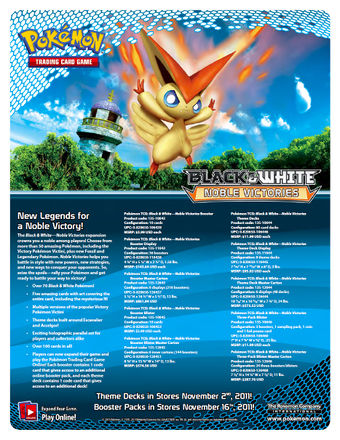The image appears to be an e-zine article or advertisement for the Pokémon Trading Card Game. The central figure is a small, yellow-and-orange Pokémon with an angry expression, emanating fire and energy. This creature has extended arms and legs, large pointy ears, and wings.

In the top left corner, the official Pokémon Trading Card Game logo is prominently displayed against a digital hexagon pattern. The header image also includes an outdoor setting with trees, sky, and a building in the background, alongside the text "Black and White Mobile Victories."

Below the main image, the header reads "New Legends for a Noble Victory," followed by three columns of text, though the fine details are hard to discern due to pixelation and JPEG artifacts. Bullet points and additional text are seen beneath these columns, indicating release dates for new products: "Theme Decks in stores November 2nd, 2011," and "Booster Packs in stores November 16th, 2011."

At the bottom, the Pokémon Company logo is positioned in the bottom right corner, while the phrase "Play Online" appears in the bottom left.